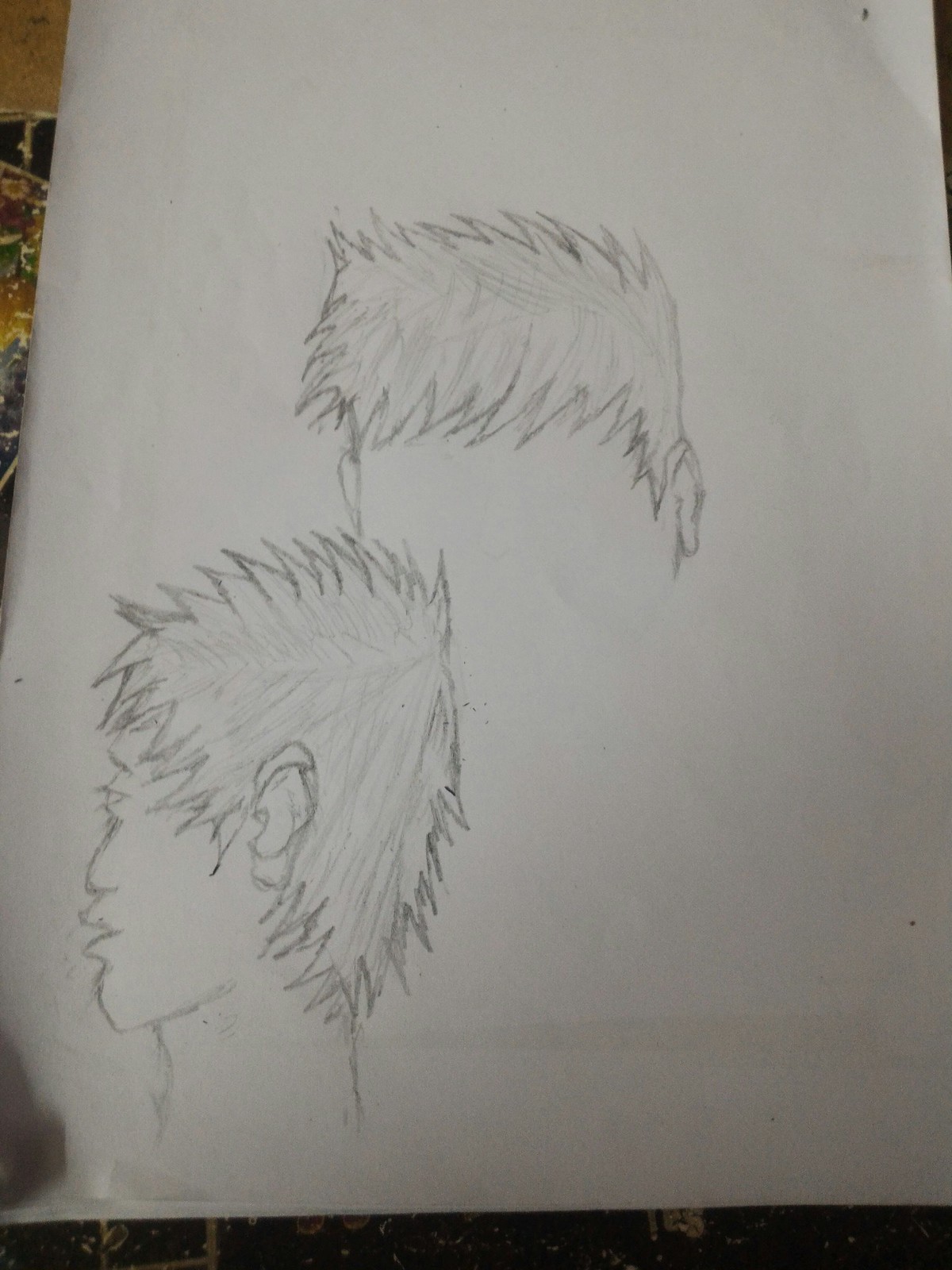This black-and-white illustration is set against a white piece of paper. On the bottom left of the drawing, there is a detailed side profile of a person showcasing their hair, ear, eye, nose, mouth, and neck. Centered in the image is another head, depicted with hair and ears but lacking facial features, presenting a blank, white face. In the background, slightly cut off on the bottom left, there is an element in brown. Behind the paper, a multi-colored background provides contrast to the monochrome drawing.